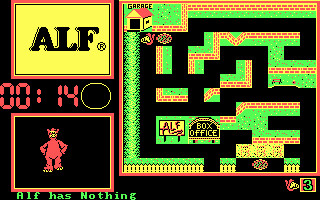The image captured is a horizontally rectangular screenshot from a video game. The background is entirely black, creating a stark contrast with the game's interface. In the upper left corner, there is a prominent large yellow box outlined in red, containing the name "ALF" written in bold black letters. Below this box, a timer is displayed in red, currently counting down from 14 seconds. 

Directly beneath the timer, another black box, also bordered in red and yellow, features a small red character identified as "ELF" (possibly a typo intended to read "ALF"). Further below, in green text, the phrase "ALF has nothing" is boldly displayed. 

Occupying the right side of the frame is the gaming area itself, depicted as a maze. The maze's pathways are illustrated in black, contrasting against the maze's intricate borders, which are colored in a vivid teal green with red brick patterns. The overall composition conveys an intense and visually compelling gaming experience, emphasizing the urgency of the countdown and the challenge presented by the maze.